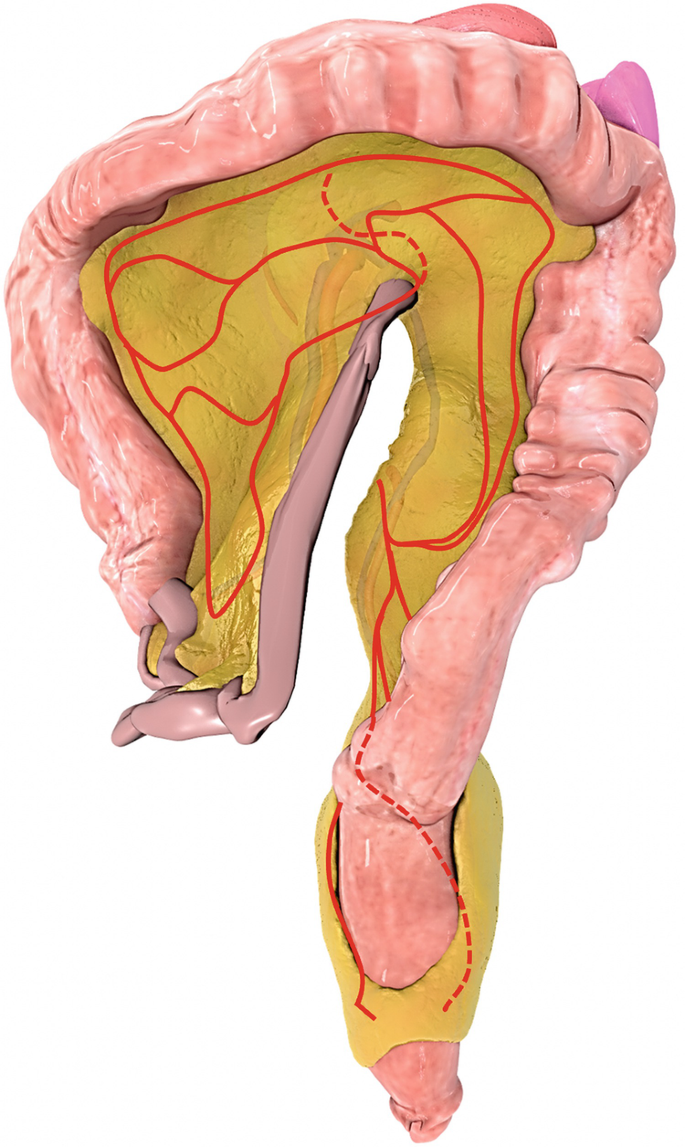The image depicts what appears to be a detailed illustration of an intestine viewed from the side. The outer layer of this organ is a pinkish flesh color, with a texture that suggests wrinkles, potentially mimicking the appearance of a colon. This pink outer layer forms a noticeable question mark shape. Beneath this outer pink layer lies a more prominent yellow interior, also following the question mark pattern. Within the yellow section, there are red and blue lines, likely representing veins or blood vessels, with the red lines transforming into red dotted lines towards the bottom of the question mark form. The yellow interior is somewhat transparent, placed against a white, transparent background. The image's clarity is high, capturing these anatomical details with an illustrative style that highlights the complexity of the organ's structure.